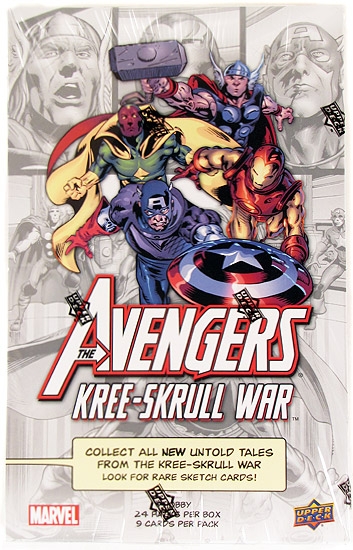The image depicts a vibrant wrapper for The Avengers trading cards from the comic book series "The Avengers: Kree Skrull War." Dominating the foreground are intricately pencil-drawn and vividly colored depictions of iconic Marvel superheroes Captain America, Iron Man, Thor, and Vision. Captain America is notably striking and robust, positioned on the lower left, while Thor, brandishing his hammer, stands prominently at the top right. Iron Man is clearly visible on the right. Positioned at the top center, the title "The Avengers" is bold in white lettering with a red outline, followed by "Kree Skrull War" in similarly styled text with a black shading and red shadowing. A beige text box near the bottom emphasizes, "Collect all new untold tales from the Kree Skrull War. Look for rare sketch cards." The background features faint, artistic pencil sketches of these heroes in various poses, providing depth to the visual. Logos for Marvel and Upper Deck are placed at the lower edge of the wrapper, signifying authenticity.